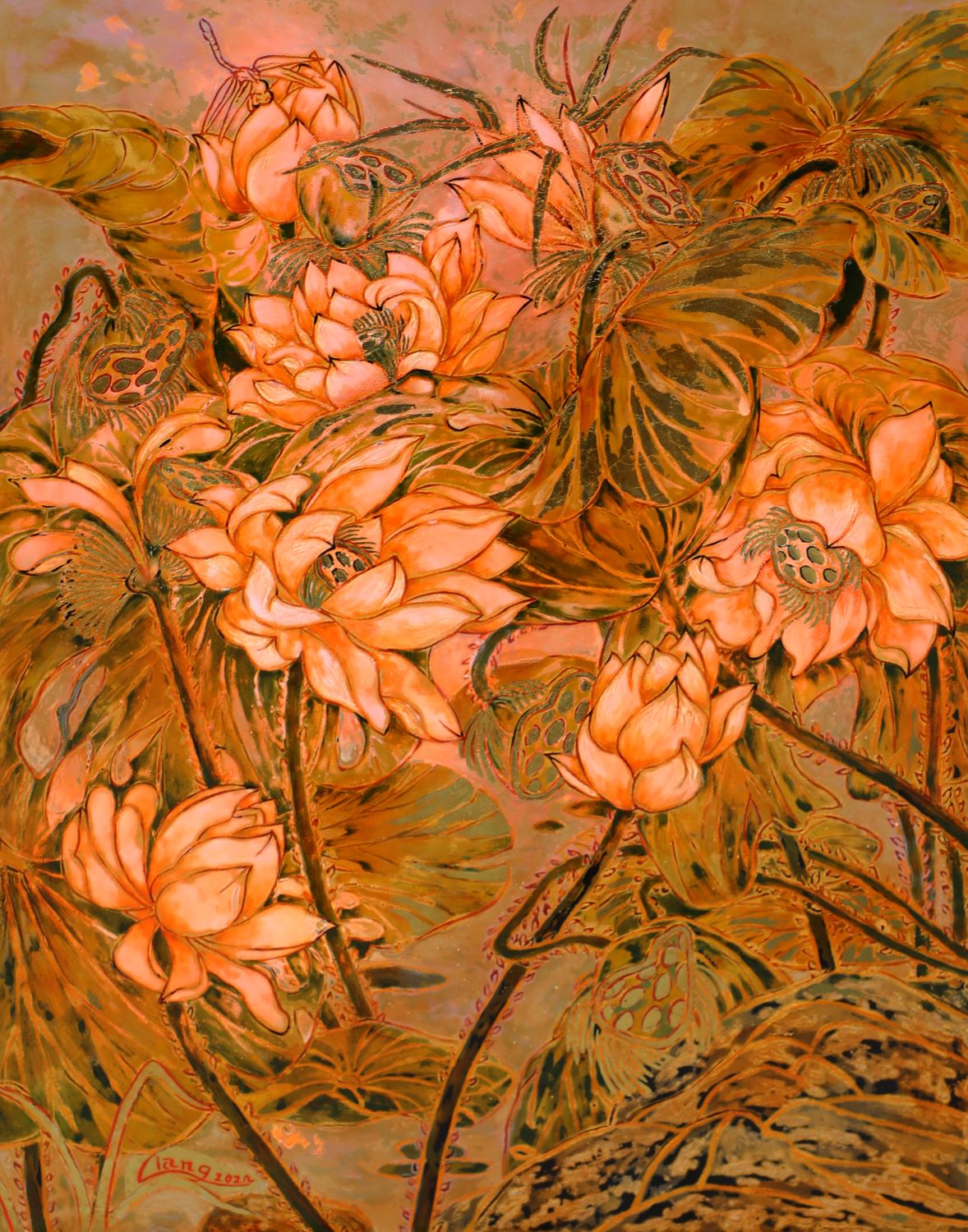This image is a color painting in a portrait orientation that intricately captures a cluster of flowers on stems with leaves around them. The painting, which resembles a photo due to its detailed and realistic appearance, features flowers spread out randomly across the canvas, creating a harmonious yet spontaneous arrangement. The flowers, multi-petaled and uniquely detailed, showcase a palette of peachy orange hues. Prominent within the composition is a large blossom curving toward the center on the left, accompanied by two smaller blooms behind it—one positioned below and the other slightly above. Additionally, three more blossoms are arranged above this central flower, with one open and facing left, another more closed and pointing upwards, and the third directed to the left. On the right side, there are two more blossoms; the central flower is facing down, while the smaller one below it is not yet fully opened. The stems, illustrated in a dark, blackish-brown shade, complement the lacy-patterned leaves rendered in brown and green tones. Layers of thread-like grass add depth to the bottom of the painting. The background is modeled and out of focus, enhancing the intricate foreground elements. The subtle details, such as individual petals and various buds, highlight the uniqueness of this work, which is created in the distinct style of a Vietnamese lacquer painting.